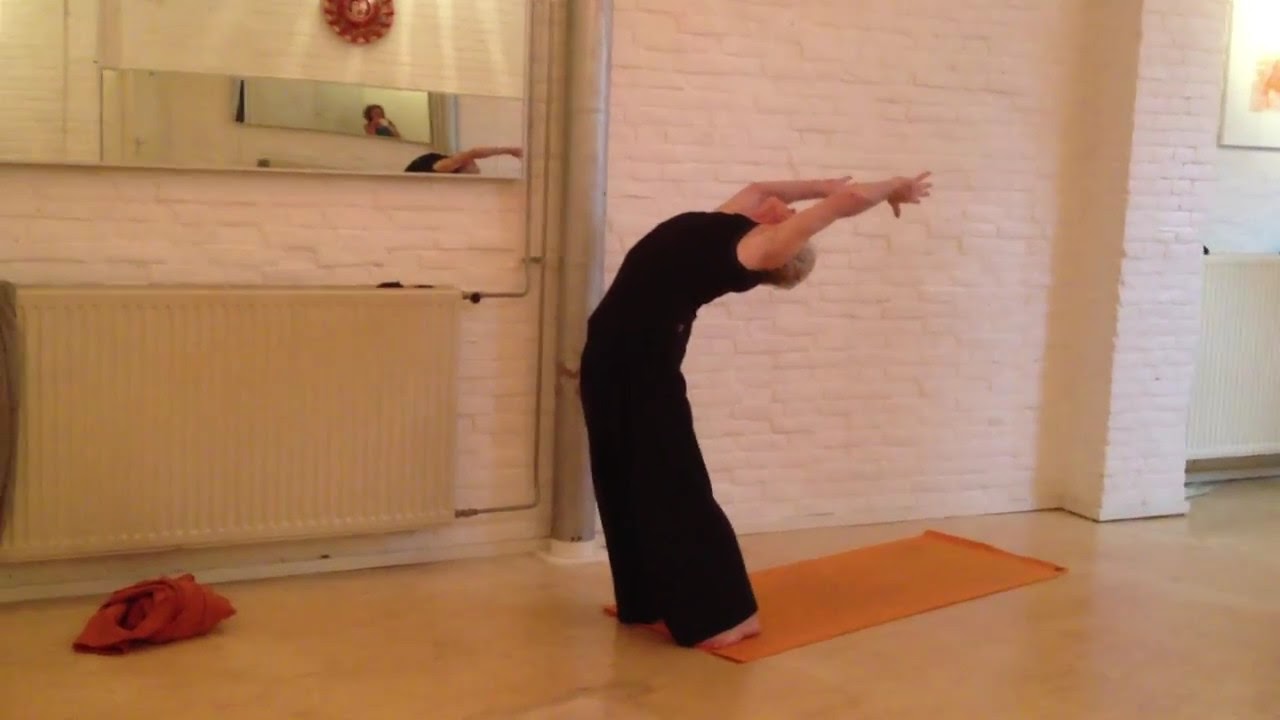The image features an older woman gracefully executing a yoga pose on a yoga mat in a quiet studio. She is bending backwards, with her waist arched and her head parallel to the floor, reaching out with both hands. The spacious studio has a bare, clean floor, possibly dampened to prevent slipping, and undecorated walls that contribute to the minimalist environment. The woman wears a black outfit, which appears comfortable and suitable for movement. In the left background, a mirror reflects her form and also shows the photographer capturing the moment. An orange bag is visible on the floor nearby, suggesting the presence of personal belongings. The serene and solitary setting hints that she might be an instructor, possibly preparing for a class or enjoying a solitary practice session.